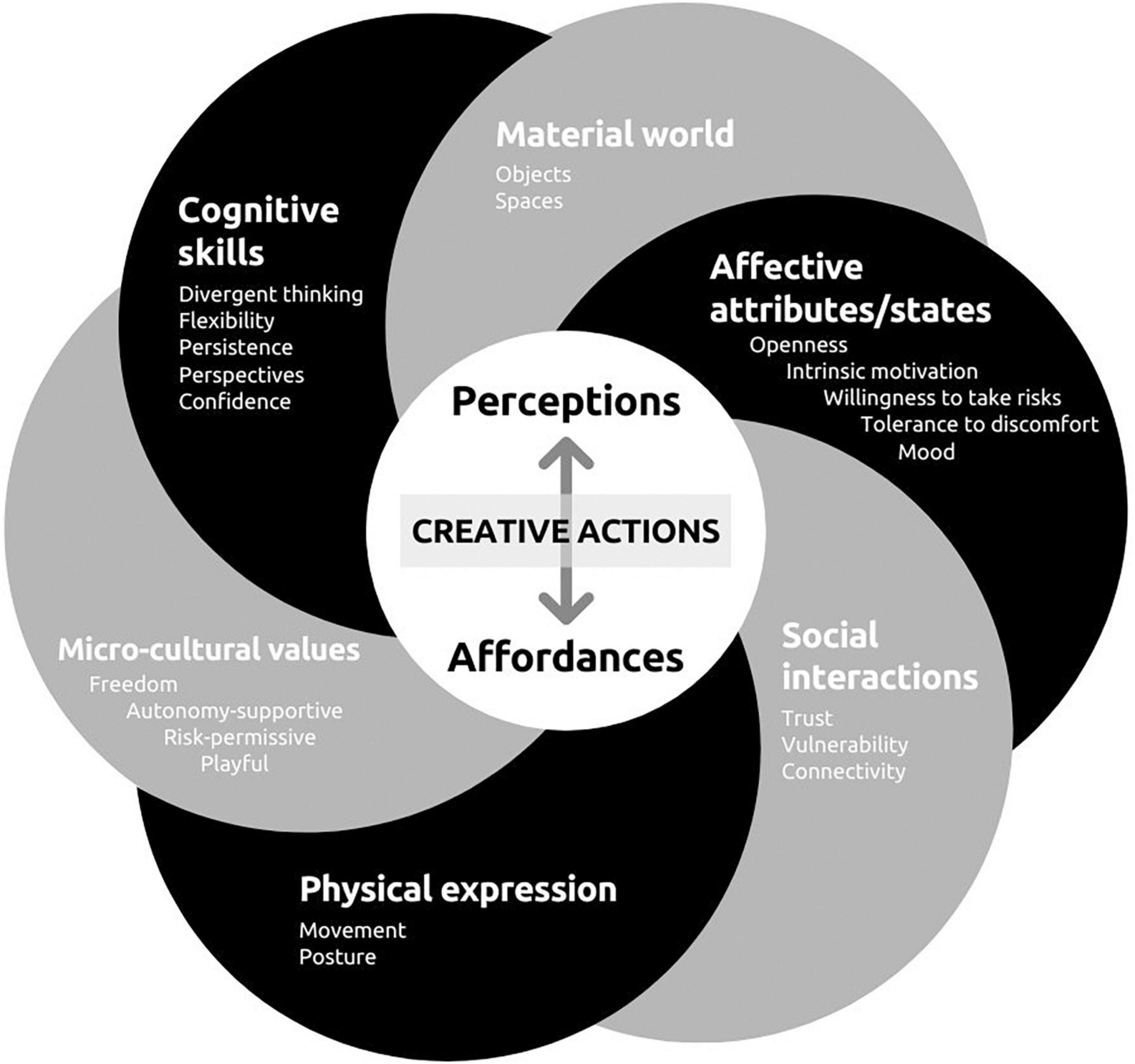The image depicts an intricate, circular infographic with a monochromatic design featuring black, white, and gray shades. At the center of the infographic, a white circle labeled "Perception" is prominently positioned, with an arrow pointing towards it. Below this primary circle, a rectangular section labeled "Creative Actions" is intersected by an arrow pointing upwards and another pointing downwards, leading to the word "Effort" at the bottom.

Surrounding the central circle, there is a series of overlapping circles that alternate between black and gray. These circles form a larger, composite circle and are each labeled with different attributes and categories. For instance, one gray circle is labeled "Material World" and includes subtexts like "Objects" and "Spaces," while a black circle next to it details "Affective Attributes and States" including "Openness," "Intrinsic Motivation," "Willingness to Take Risks," and "Mood."

Additional gray and black circles provide further categorization: "Social Interactions" (with subtexts "Trust," "Vulnerability," and "Connectivity"), "Physical Expressions" (with "Movement" and "Posture"), "Microculture Values" (emphasizing "Freedom," "Autonomy," and "Supportiveness"), and "Cognitive Skills" (listing "Divergent Thinking," "Flexibility," "Persistence," "Perspective," and "Confidence"). Each of these categories is detailed in white text, enhancing readability against the alternating backgrounds. This infographic effectively conveys complex interrelations among cognitive, physical, social, and cultural factors in a visually engaging and organized manner.